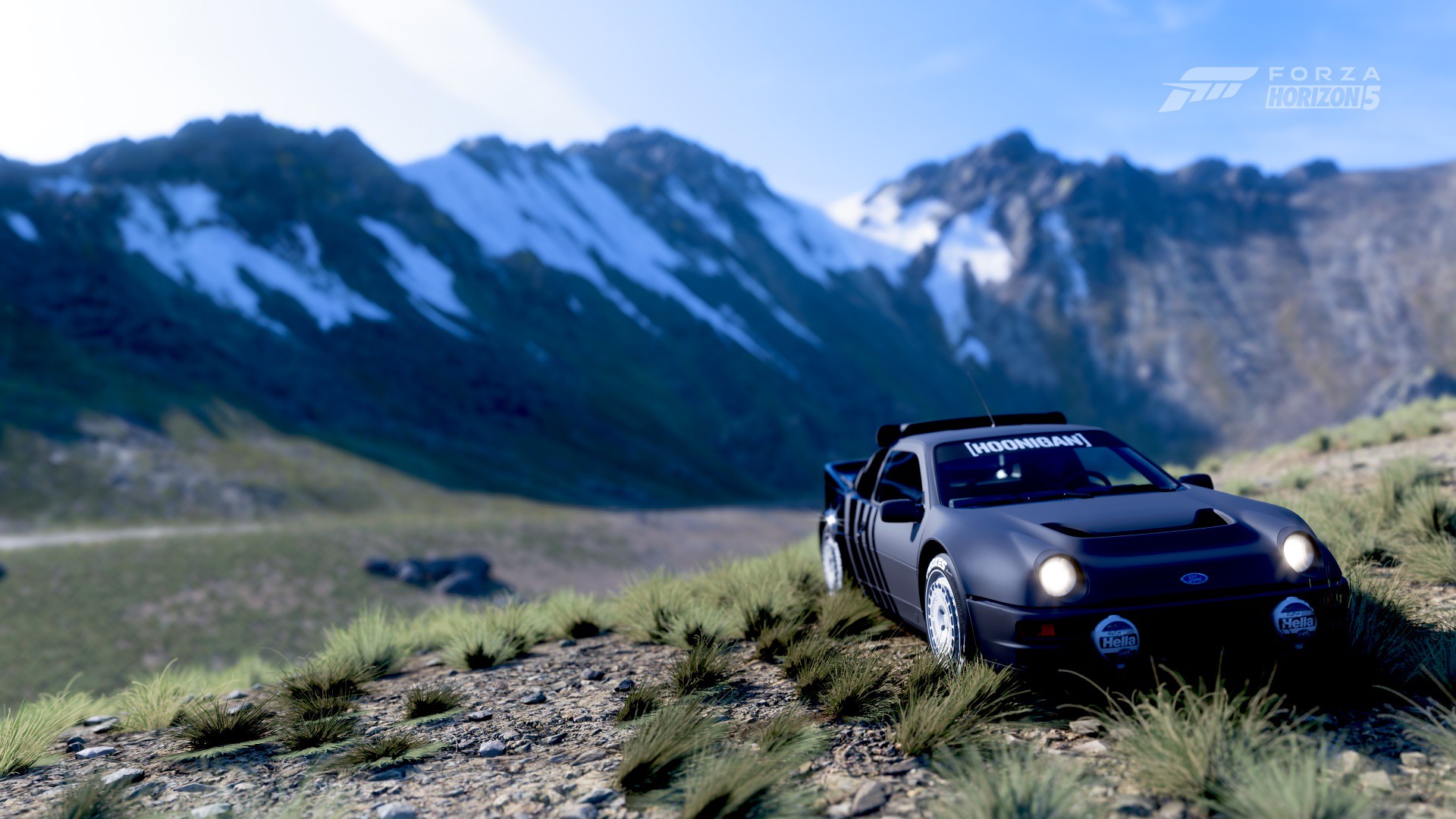In this detailed and digitally-rendered scene, a sleek silver Ford sports car, bearing the bold white lettering "H-O-O-N-I-G-A-N" on its windshield, is prominently displayed in the foreground. The car's headlights are illuminated, adding a pop of brightness against the natural backdrop. It sits parked on a mix of soil and low grass, with two front portals covered in a conspicuous red and white design that says "hello." Dominating the background is a stunning range of snow-capped mountains, their peaks casting shadows over a serene valley below, all beneath a clear, blue sky. The upper right-hand corner of the image proudly displays the watermark "F-O-R-Z-A Horizon 5," indicating that this is a screenshot from a video game. The scene is enhanced with a unique graphic element of slanted, tape-like rectangles adding an artistic touch to the composition.